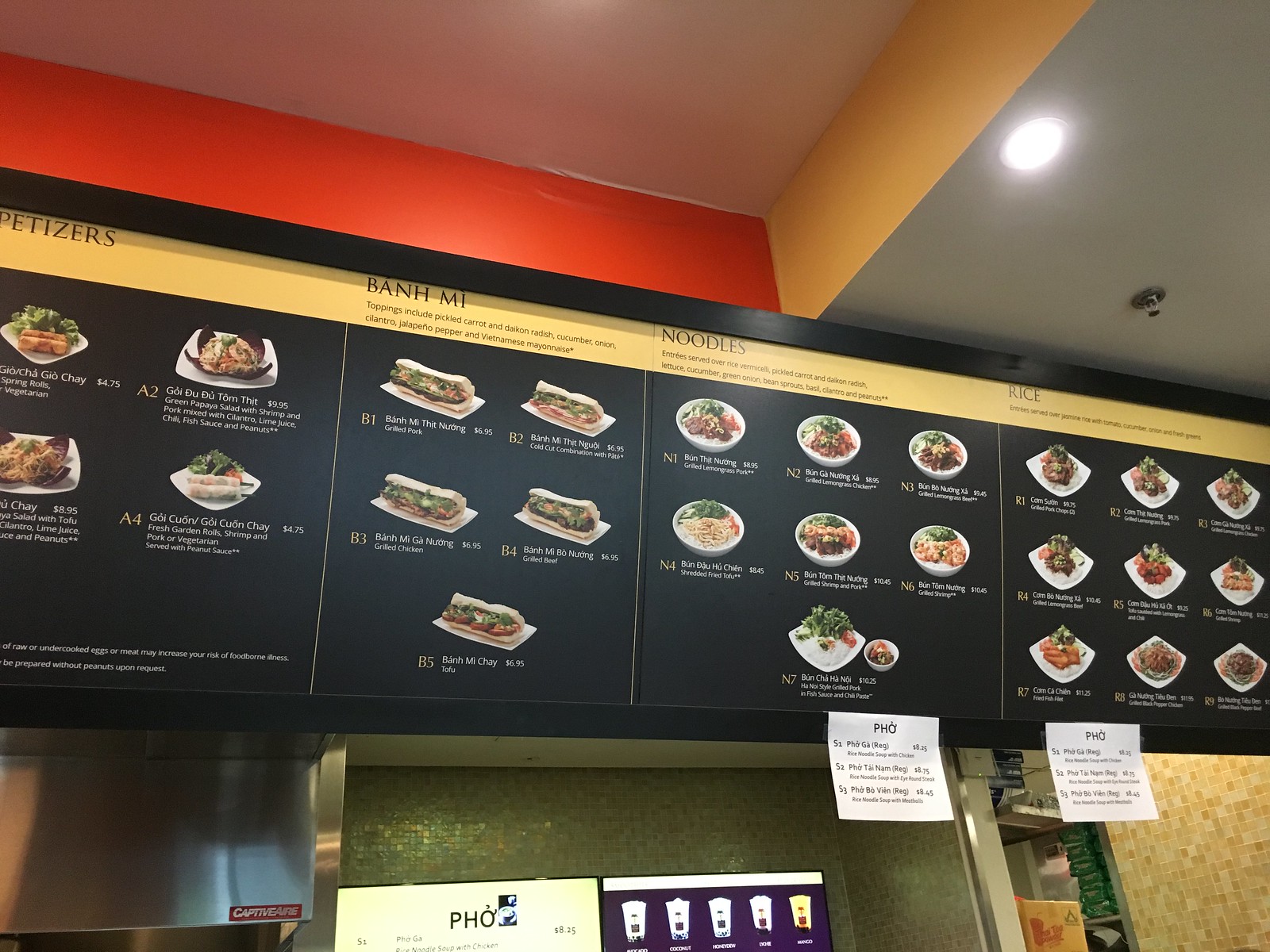This detailed caption describes the image:

"The image features a detailed menu set against a black background. On the right side of the menu, there is a section dedicated to noodles, followed by a section for rice, which includes nine different varieties. The appetizer section showcases four visible dishes, while the main section offers a selection of five dishes that include sandwiches and noodles. Additionally, there are six bowls and one square bowl arranged in the depiction of dishes.

In the background, the top left corner of the image shows walls painted in red, while the top right corner is accented with yellow. The ceiling has a touch of white, and there are white accents on the right side as well, along with visible sprinklers. Numerous stickers displaying Pho indicate that this is an Asian restaurant. At the bottom of the image, a variety of drinks are presented, adding to the detailed layout of this vibrant and inviting menu display."